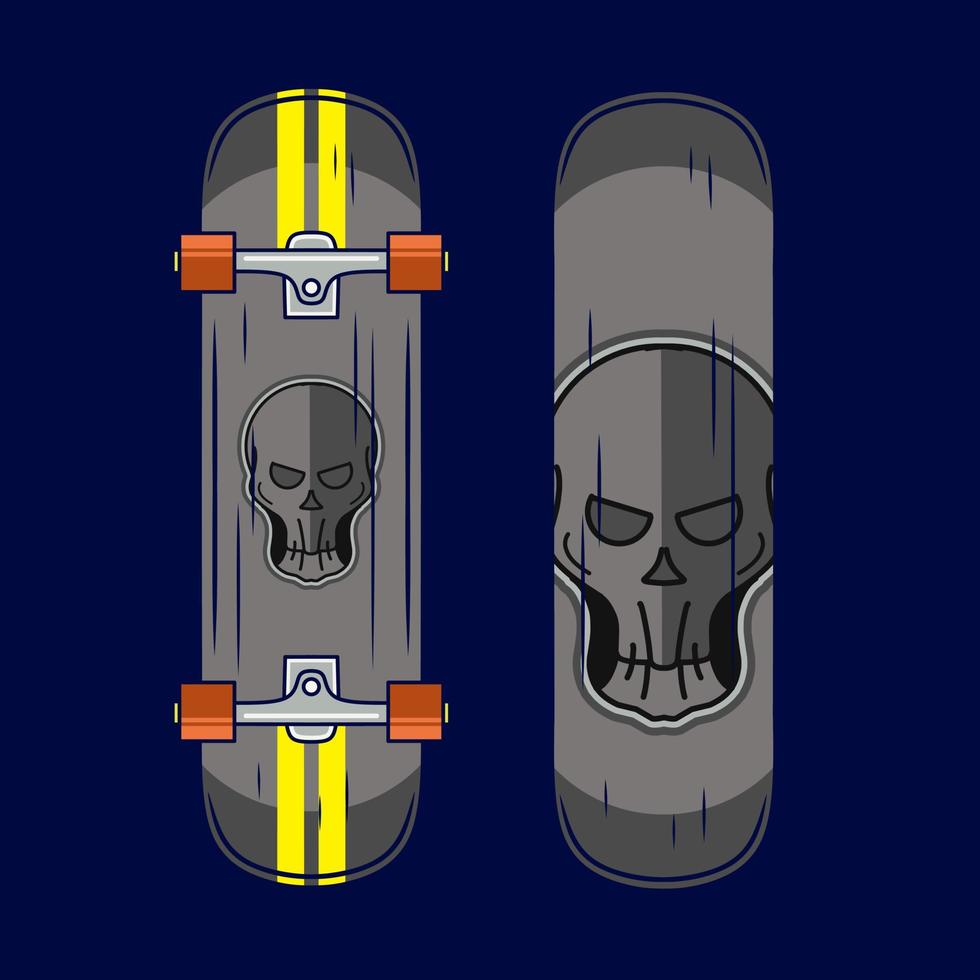This detailed drawing features a vertically rectangular image with a dark blue background and no border. The image showcases two skateboards, positioned one on the left side and one on the right side. The left skateboard displays the underside, revealing metallic struts for the wheels, which are orange. Two vertical yellow lines extend from the center of the metal rod, reaching both the top and bottom of the skateboard. Centered on this side is an artistic depiction of a skull. The right skateboard presents the topside, characterized by a plain gray surface that's darker at the top and bottom, and lighter in the middle. It also features a larger version of the same skull design. The overall color scheme includes mostly gray tones with accents of yellow and orange, set against the dark blue background.